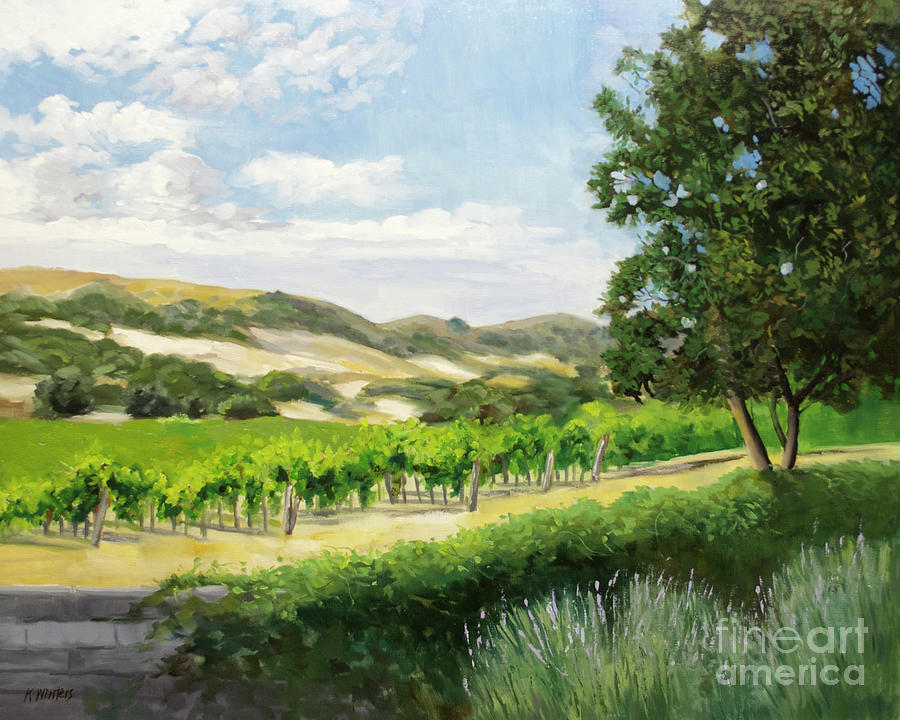This detailed landscape painting, possibly done in oil or acrylics and signed by K. Winters, features a serene outdoor scene marked by a vivid blue sky adorned with white, puffy clouds. Dominating the foreground is a stone wall lined with a hedgerow and tufts of various grasses and plants, possibly cattails. To the immediate right, a tree in full foliage frames the view. Spanning the midground are what appear to be meticulously organized rows of grapevines or fruit trees, suggestive of a vineyard or orchard. These rows are supported by a series of fences, leading into a gentle valley below. Surrounding this cultivated area are rolling hills, some parts of which are arid and sandy with interspersed greenery. A mysterious gray structure is faintly visible on the left side. The painting also contains green bushes and trees, adding to the lushness of the landscape. A semi-transparent watermark reading "Fine Art America" is situated in the lower right corner.